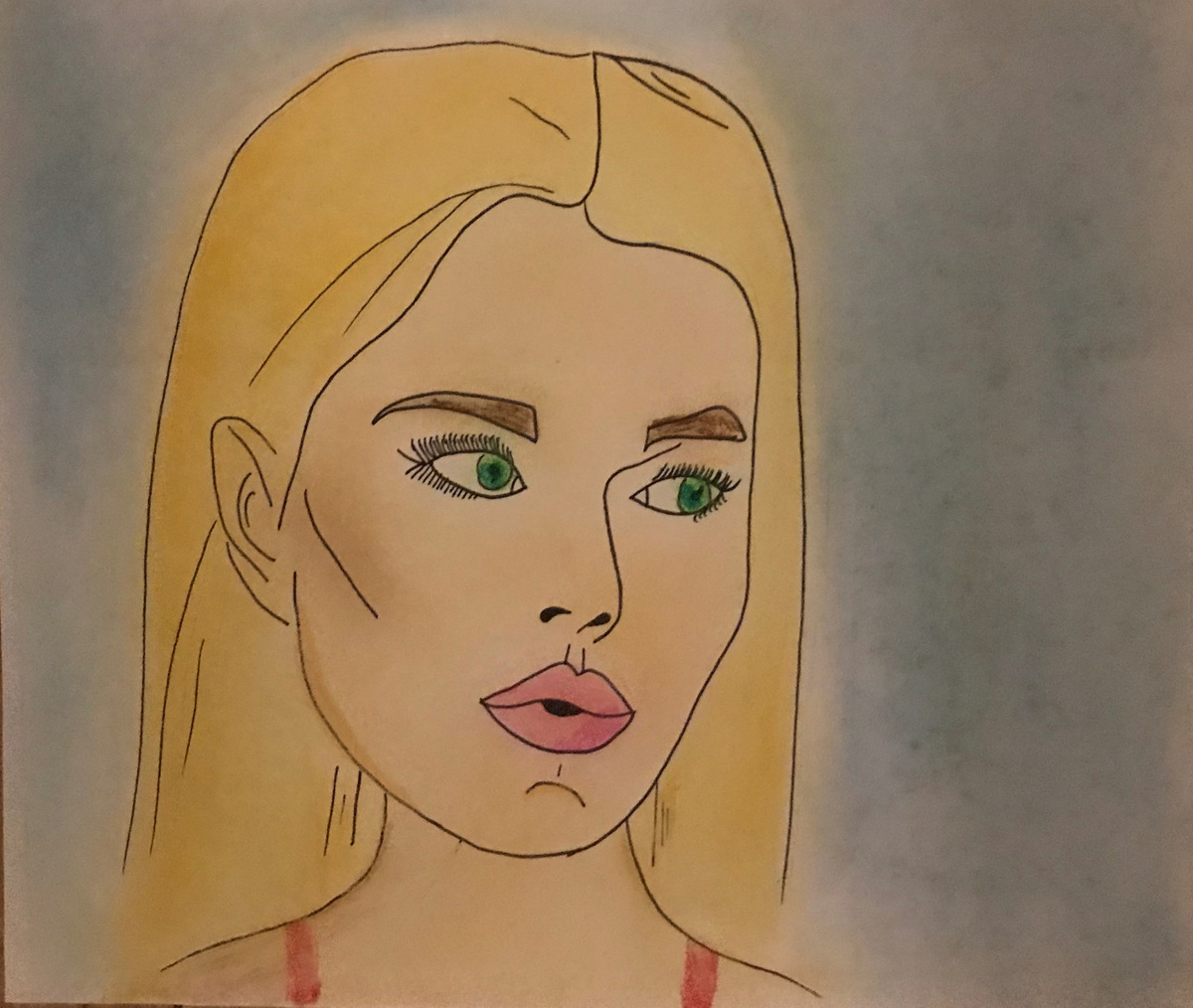This detailed colored pencil sketch captures a close-up portrait of a young white woman with shoulder-length blonde hair, parted neatly in the middle. Her striking green almond-shaped eyes are adorned with thick eyelashes and defined, full eyebrows. She has a pointy nose and soft, pouty pink lips, adding to her expressive features. A cleft chin and an exposed left ear further characterize her unique appearance. Her straight blonde hair frames her fair complexion, and she is depicted wearing a red tank top, with just a hint of the straps visible. The background is a very light blue, enhancing the portrait's overall subtlety and charm. The sketch is rendered on a piece of paper, showcasing an artist's meticulous attention to detail.